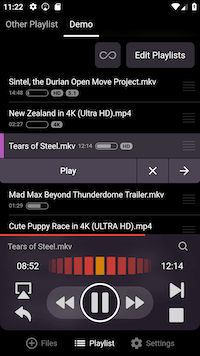The image depicts an interface of a musical app, showcasing various playlists and media options. At the top, the time is displayed as 11:22, accompanied by tiny icons for settings and battery percentage.

Below the top row, there are tabs labeled "Other Playlists" and "Demo," with the user currently viewing the demo page. Directly beneath, an infinity logo and an "Edit Playlist" option are present. 

The main content section lists various media items, starting with "Sentinel: The Durian Open Move Project" in MKV format priced at $14.48. Following this is a file labeled "New Zealand in 4K Ultra HD" in MP4 format. Next is "Tears of Steel" in MKV format, priced at $12.14.

Below these items, playback controls are displayed. There is a "Play" button, an "X" to close, and a right-pointing arrow. 

Further down, "Mad Max Beyond Thunderdome Trailer" in MKV format is listed, with a run time of 1 minute and 29 seconds.

At the bottom of the list, the currently playing item is "Cute Puppy Race in 4K Ultra HD" in MP4 format, showing that .852 of 12 minutes and 14 seconds has been played. Control symbols for pause, and left and right arrows are also visible.

Finally, the bottom navigation bar includes three options: Files, Playlists, and Settings.